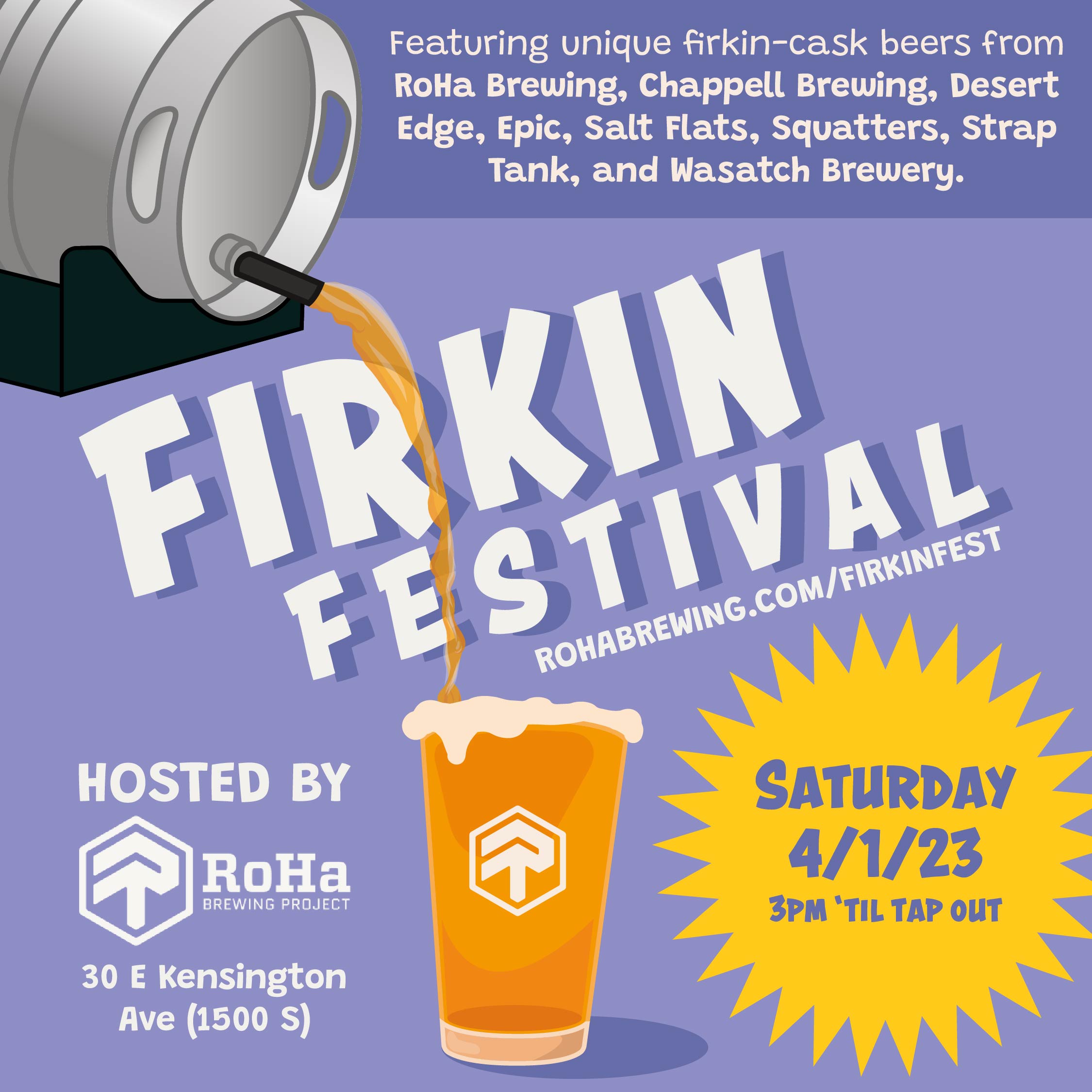The image is a digitally generated beer festival advertisement with a predominantly gray or blue background. In the top left corner, there is a cartoon illustration of a silver beer keg, which is pouring beer into a pint glass positioned in the bottom-center of the image. The text is overlaid in white, with some notable sections in blue and gold. A prominent yellow sun emblem with spiky triangles is located in the bottom right corner, containing blue text. The middle of the image features large diagonal letters reading "Firkin Festival." Additional text around the image includes details about the event: "Saturday, 4-1-23, 3 PM till tap out" and "Hosted by Roja Brewing Project." The event will feature unique firkin cask beers from various breweries, including Roja Brewing, Chappelle Brewing, Desert Edge, Epic, Salt Flats, Squatters, Strap Tank, and Wasatch Brewery. The address provided is 30 East Kensington Avenue. The colors throughout the advertisement are dark blue, light blue, white, gold, gray, black, yellow, and pastel purple.